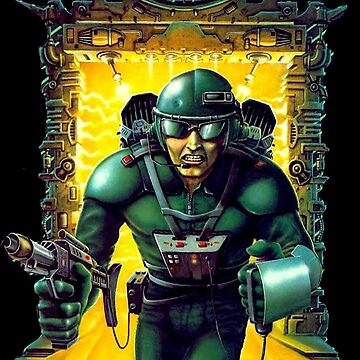The image is a highly detailed, color illustration of a futuristic fantasy soldier, depicted as a male character in a tight-fitting green bodysuit, helmet, and green tinted sunglasses which obscure his eyes. The soldier's expression is fierce, with a scowl and gritted teeth, radiating determination as he faces the viewer. In his right hand, he holds a futuristic laser gun, which is connected to a box on his tool belt by a cord. His left hand wields an enigmatic, round object that resembles brass knuckles or a small shield. The soldier also dons black gloves, and a complex apparatus on his chest, possibly a battery or control unit, adorned with numerous flashing lights. Additionally, he appears to carry a jetpack on his back. The background features a mechanical doorway, framed by intense yellow light and flames, contrasting against the predominantly black backdrop, creating a dramatic and dynamic scene.